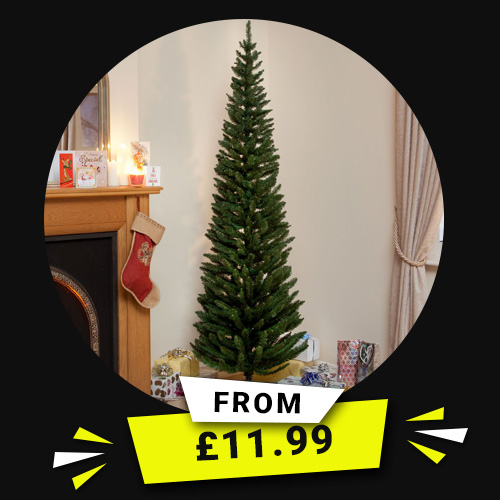A festive photograph captures the cozy ambiance of a holiday-decorated room. Dominating the scene is a slender Christmas tree adorned with simple decorations, situated against a beige wall. The square photo is artfully framed with a circular vignette effect, drawing attention to the tree at the center. Underneath the tree, a variety of wrapped presents add a touch of holiday cheer.

To the right side of the image, a window dressed in elegant draperies, tied back to reveal a hint of the outside, enhances the room's warm and inviting feel, though the view outside is not discernible. On the left, a wooden fireplace mantle acts as a backdrop, graced with a single, vintage-looking stocking. A collection of Christmas cards rests on the mantle, adding to the festive decor, while above it hangs what appears to be a mirror, though its full form is partially obscured by the vignette framing.

At the bottom edge of the image, two trapezoidal shapes in black and yellow respectively provide a quaint touch, the white one labeled "From," and the yellow announcing "11.99 pounds," suggesting that the Christmas tree is available for purchase at a price just under twelve pounds. The overall composition encapsulates the warmth and simplicity of the holiday season.